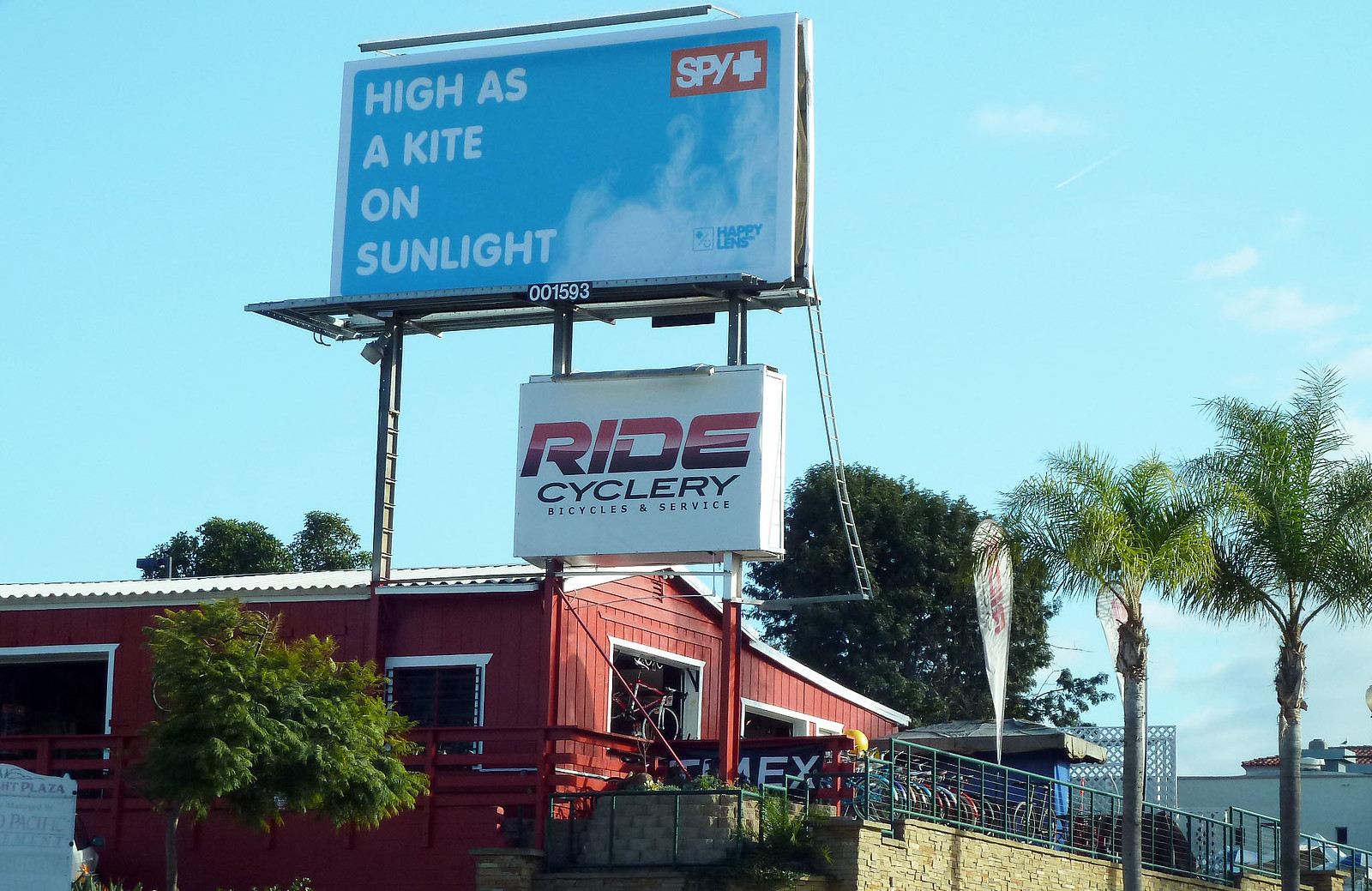The image depicts a quaint, old-fashioned bike shop nestled on a sunny beach, likely located in either Florida or California. The shop, named "Ride Cyclery, Bicycles & Service," is an eye-catching red structure with white trim and a white roof, resembling a classic barn. Constructed from wooden panels, the shop exudes a rustic charm. Through the open front, a variety of bicycles are visible inside.

Prominently displayed on the front of the shop are two large signs. One bears the shop's name and services, while the other, a bulletin board, features the quirky message: "High as a Kite on Sunlight, Happy Lens, Buy Plus, 0015938." The exterior scene is completed by a porch where an array of brightly colored bicycles are neatly lined up.

Surrounding the shop are two tall palm trees on the left and several other trees, accentuating the beachside setting. The ocean is visible in the background, adding to the serene coastal vibe. The sky is clear and sunny, with minimal clouds, suggesting perfect beach weather. A villa can be seen in the distance, enhancing the picturesque scenery.

In front of the shop, a faded sign reads, "Something Plaza, Pacific," with the last part too worn to decipher, suggesting that this charming bike shop could indeed be located along the Pacific coast, likely in California.